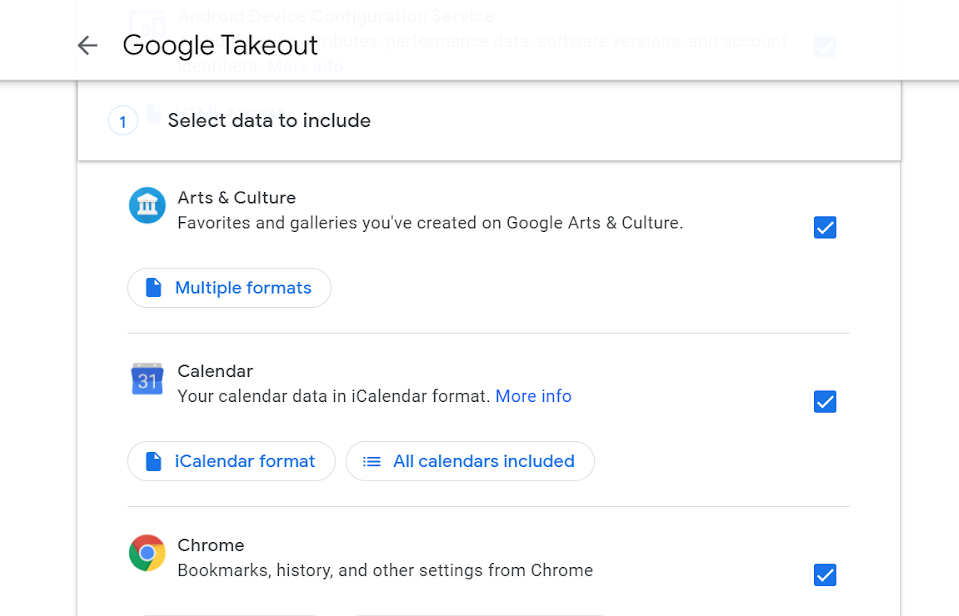In this image, we see a screenshot of the Google Takeout interface. At the top, there is a black and white header displaying the text "Google Takeout" alongside a leftward-pointing arrow, presumably a back button. Below this header, in bold black text on a white background, it says "Select data to include." 

The first selectable option is labeled "Arts & Culture" with the description "Favorites and galleries you've created on Google Arts & Culture." This option has a blue checkbox indicating it is selected. Accompanying this selection, the text "Multiple formats" is displayed beneath it. 

Moving down, the next selectable option is "Calendar," identifiable by its calendar icon. It states, "Your calendar data in iCalendar format. More info." Like the previous option, this also has a blue checkbox indicating it is selected. Underneath, it specifies, "iCalendar format and all calendars included."

Further down, the final option visible is "Chrome," marked with the Chrome icon. It describes, "Bookmarks, history and other settings from Chrome," with a blue checkbox next to it, indicating selection.

The entire interface is designed with a clean, white background, making the black text highly readable.